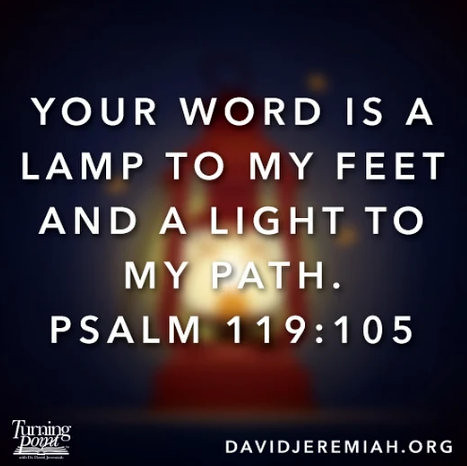This social media graphic features a vivid motivational Bible verse set against a dark, blurry backdrop that highlights a red handheld lantern. The lantern is situated centrally, casting an illumination that creates a star-like effect around it, enhancing the image's mystical ambiance. Dominating the center of the graphic, large bold white text proclaims the verse, "Your word is a lamp to my feet and a light to my path, Psalm 119:105." The lower left corner displays the Turning Point logo, while the bottom right contains the URL davidjeremiah.org, directing viewers to additional resources.